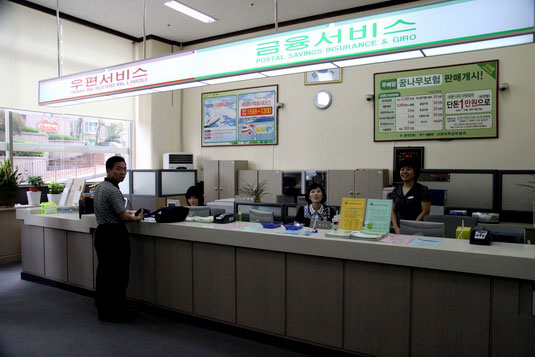The image depicts the interior of an Asian, possibly Japanese or Chinese, postal office. Three female postal employees stand behind a gray countertop, equipped with computers and a phone. The employee on the far right is noticeable for her dark shirt and friendly smile. Engaging in business at the counter is a man who has turned to face the camera. To the left of the scene is a large window offering a view of the street outside. The floor inside the post office is blue. Above the counter, two large signs with Asian writing hang on the wall; one sign is blue and white, while the other is green and white. Additionally, there are various colored posters and flyers — including red, green, blue, and yellow — decorating the space. This detailed setup suggests the establishment functions as a postal office with banking and insurance services.